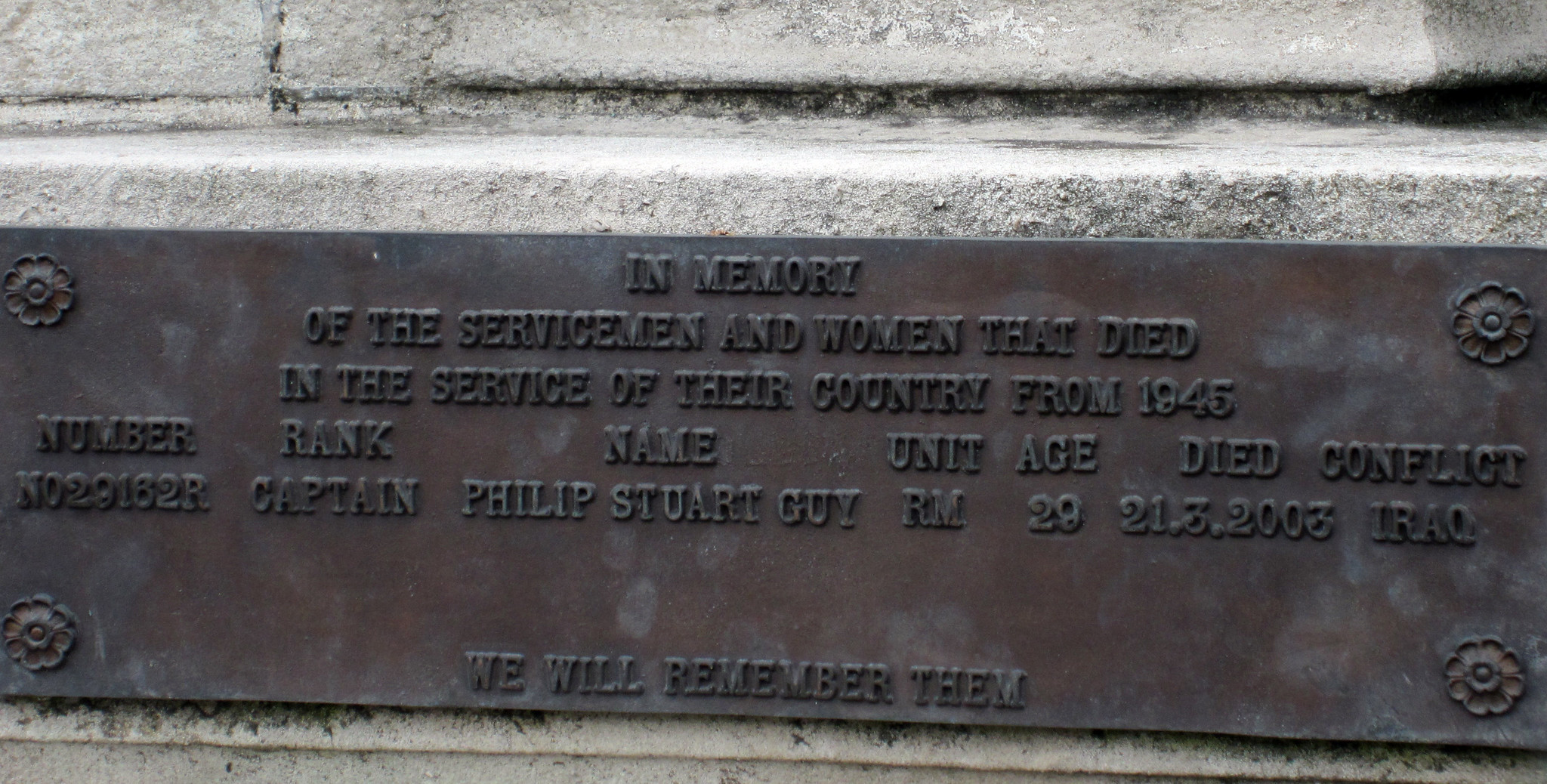The image showcases a memorial plaque affixed to the white stone base of a monument, which gradually narrows towards the top. The dark brown, rust-colored plaque is adorned with decorative florets in each of its four corners. This plaque commemorates servicemen and women who died in the service of their country since 1945. Prominently displayed is the inscription, "In memory of the servicemen and women that died in the service of their country from 1945." Below this dedication are columns listing the service details. The singular entry reads: "Number: N029162R, Rank: Captain, Name: Philip Stuart Guy, Unit: RM, Age: 29, Died: 3-21-2003, Conflict: Iraq." At the very bottom, a solemn tribute, "We will remember them," concludes the inscription. Small flowers can be seen at the left and right corners of the plaque, adding a touch of nature to the somber memorial.